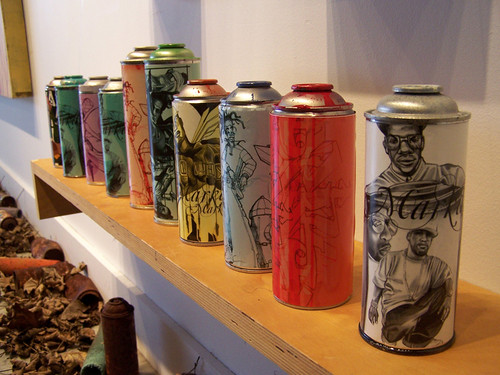The photograph depicts a wooden shelf mounted against a white wall, holding a line of ten spray paint cans. Each can is personalized with intricate and artistic illustrations, including drawings of people and various graffiti-style designs. The cans, which vary in color and size, notably lack their spray nozzles. To the bottom left of the image, there is a collection of discarded, rusted spray paint cans surrounded by dirt, debris, and trash, adding a stark contrast to the clean surface of the shelf. This scene suggests an art installation, blending the aesthetics of the displayed cans with the chaotic, discarded ones below.